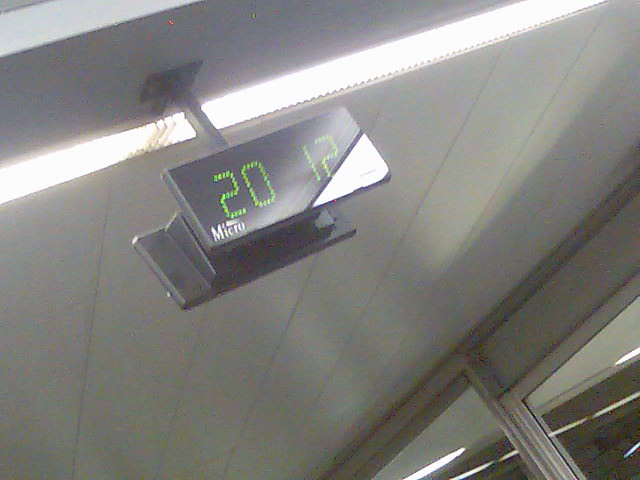The image depicts a slightly askew, blurry interior scene likely set in an airport or train station, characterized by bright, strip fluorescent lighting. Hanging from the plain, white, line-patterned ceiling is a two-faced rectangular electronic LED sign displaying the numbers "20" and "12" in green, dot matrix-style numerals. This sign, suspended by a bar bolted to the ceiling, also features the word "Micro" faintly visible on the bottom left, possibly indicating the brand. The lower right corner shows the tops of two windows with reflected lights, further adding to the indoor, possibly commercial ambiance.